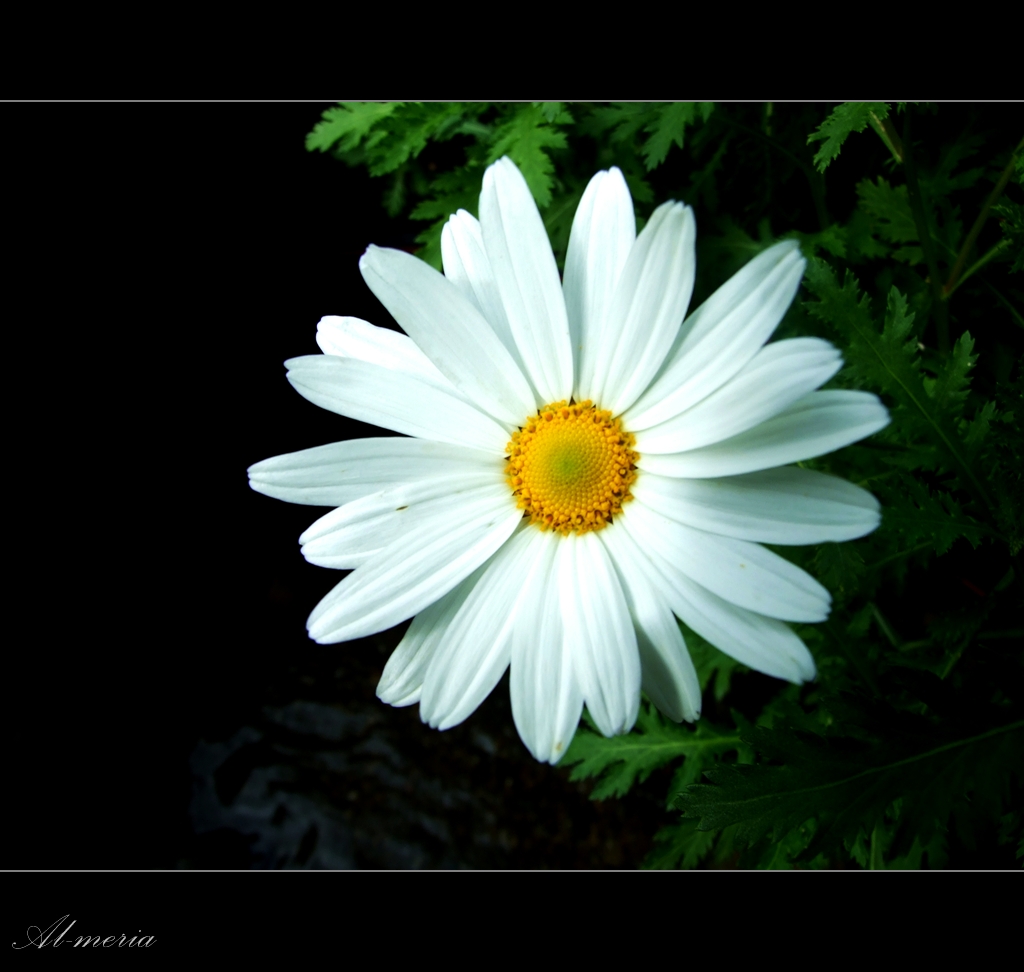A close-up photograph of a large white daisy-like flower featuring two rows of delicate, long white petals encircling a vibrant golden-yellow center that spirals down into a subtle green core. The flower is centrally positioned against a predominantly dark background, suggesting the image was taken at night with a flash to highlight the flower’s details. Surrounding the flower, faint outlines of green leaves are visible, predominantly at the sides and top of the image, contrasting against the black backdrop. The photograph is bordered by thin gray lines at the top and bottom, and in the lower-left corner, the text "Al / Mariah" appears in white italics. The stark contrast between the bright flower and the dark background effectively captures the beauty and intricate details of the flower.